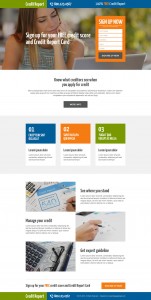The image is quite blurry, but here's a detailed description based on what can be discerned:

At the top of the image, there is a border that transitions from green to blue. The green part contains some text in white font, though the words are not legible. Similarly, the blue section also has white text that is unreadable.

In the central part of the image, there is a lady who appears to be facing the viewer. Her hair is brownish at the top, blending into a dirty blonde color as it progresses down. She is wearing a sleeveless shirt, which features a dark pattern that might consist of gray and white stripes or squares.

An overlay of white text partially obscures her face. Although the first word is unclear, the subsequent words seem to include "up for" and possibly "card." Next to this text is an orange rectangle with white text, which likely reads "Sign Up Now."

Beneath this, there are white rectangles that appear to be input fields for personal information. The background below these fields turns white and features numerous black text lines, though the exact contents are illegible. Further down, there is a dark gray rectangle containing some white elements.

On the lower portion of the image, additional elements include a picture of a calculator and glasses, as well as a hand drawing. However, the accompanying text is not distinguishable.